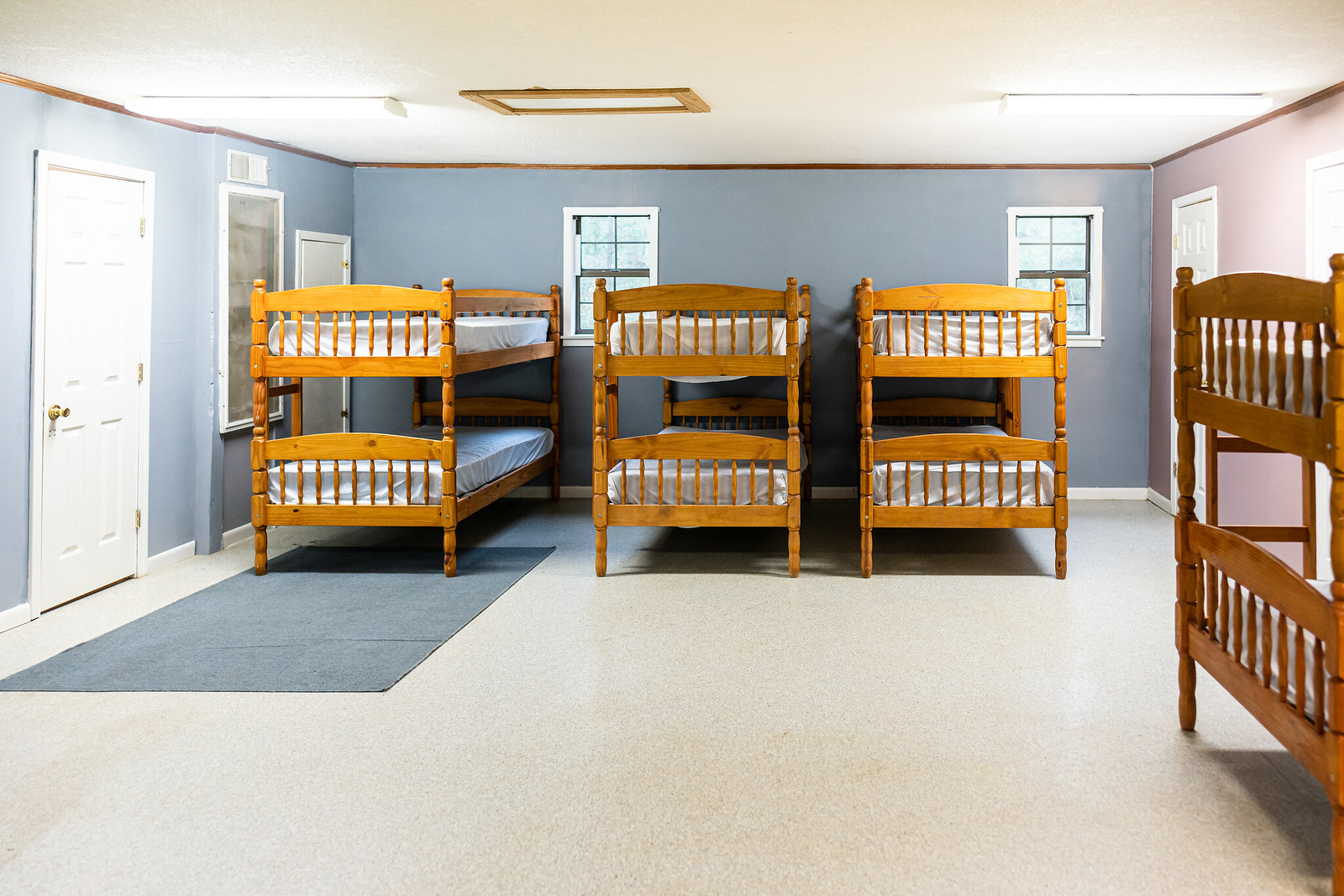The photograph captures a large indoor room with a distinctive color scheme and an arrangement of bunk beds. The back wall, painted a bluish-gray color, features two windows with white frames, allowing natural light to filter in. Below these windows, three wooden bunk beds with medium brown frames and white sheets align lengthwise against the wall. Another door, with a gold handle, is on the left side wall, which is also painted the same bluish-gray hue. On the right-hand side of the image, a pink-painted wall stands out, with a single wooden bunk bed extending outward into the room. There is also a large blue rug underneath one of the bunk beds. The room has a light gray cement floor and a white ceiling, creating a spacious and airy feel. Additionally, on the blue wall, there is a poster next to the two windows, adding a subtle touch of character to the room.